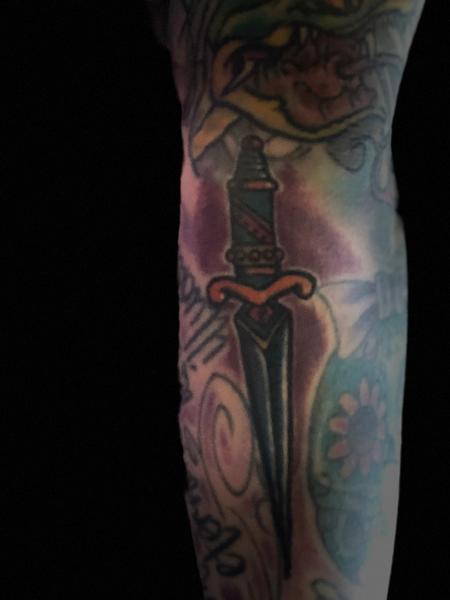The image displays a close-up of an extensively tattooed limb, likely the lower leg, set against a solid black background. The focal point is an intricate, downward-pointing dagger tattoo, located centrally on the back of the calf. This dagger features a silver blade, a gold hilt, and a handle adorned with green and red, or greenish-blue, details including a band of beads. The handle terminates with a round ball. Surrounding the dagger, the tattoo extends with various designs that include florals such as a sunflower and daisies, set against greens, and detailed shading with maroon and auburn hues. The overall tattoo composition is highly ornate and covers the entire visible area, including additional elements like writing and scroll work on the left side.